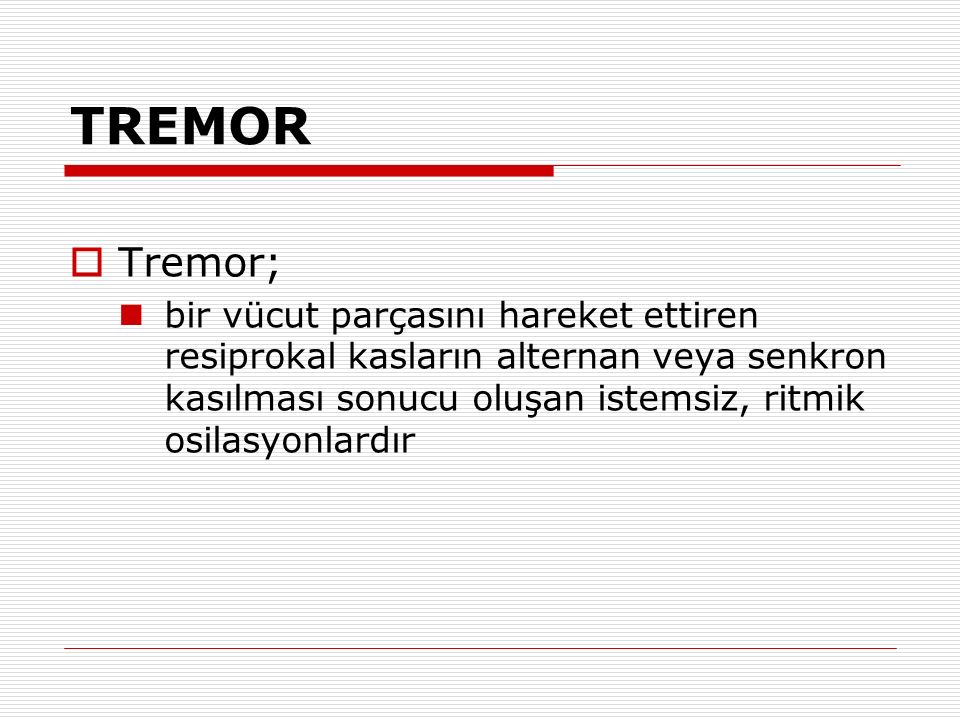The image features a sign with a heading and accompanying text, all in a foreign language. The heading prominently displays the word "TREMOR" in uppercase black letters, underlined by a thick red line which transitions into a thinner red line extending to the right. Directly below the heading, there is a small red-outlined square followed by the word "TREMOR" in a lighter font with a semicolon. Further down, there's a solid bullet point beside the text which reads: "Burr, located by Cassidy, Harrod, Kett, and Tarrant. Respiroque, castorine, alternate, VA, saccharine. Casu, mazi, sonica, odacine. Istem, zist, red milk. Orsila, ziona, dia." The overall arrangement appears as though it is providing a detailed explanation or definition, possibly scientific or medical, but the exact meaning is unclear due to the foreign language.